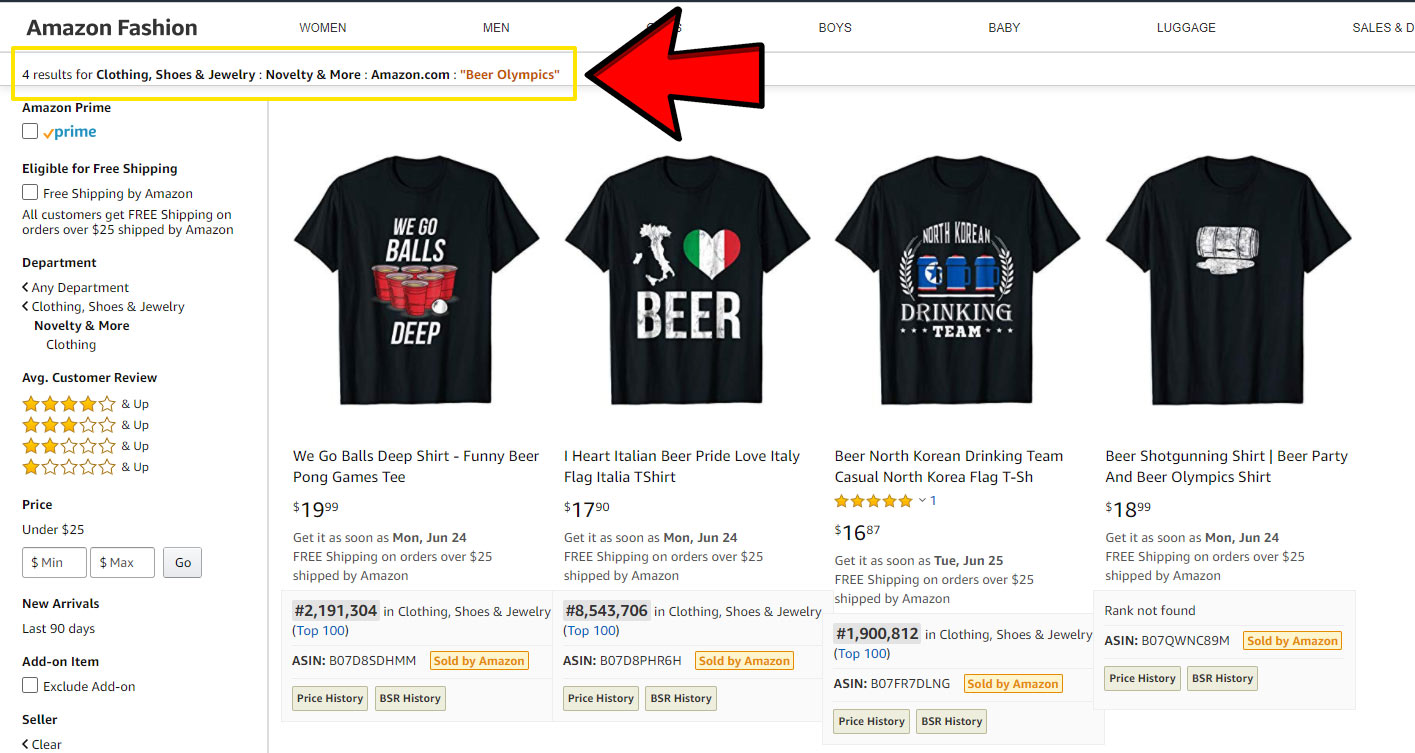### Detailed Caption 

The image falls under the *fashion* category and is set against a stark white background. Various font colors are utilized, though black predominates. At the top of the image, a black line runs across, followed by the text "Amazon Fashion." Below this, a horizontal menu lists categories: Women, Men, Boys, Baby, Luggage, Sales.

Descending the page, a striking red arrow outlined in black directs attention to a gold-bordered box, which reads: "4 results for clothing, shoes, and jewelry. Novelty and more, amazon.com." The category specified in bold red text is "Beer Olympics."

On the left side, a sidebar menu features various filters and options in black font. The top of the sidebar highlights "Amazon Prime," indicated by a white box with a gold checkmark and the word "Prime" in blue. An additional note explains that all customers receive free shipping on orders over $25 if shipped by Amazon. Below, there is another white box next to "free shipping," but it is unchecked.

Further along, the sidebar menu categorizes various departments like "Any Department," "Clothing, Shoes, and Jewelry," and "Novelty and More." Below these, filters for average customer reviews range from one to four stars. A price filter shows "Under $25," accompanied by empty boxes for setting a minimum and maximum price, with a "Go" button beside it. Additional options include "New Arrivals," "Last 90 Days," "Add-on Item," and "Exclusive Add-on," though none are checked. The section ends with "Seller" and a clickable "Clear" button next to a back arrow.

The main content displays four black shirts with various colorful graphics and text:

1. **Wego Balls Deep Shirt**: 
   - **Design**: Features the text "Wego Balls Deep" in white, alongside red solo cups and a white ping pong ball.
   - **Title**: "Wego Balls Deep Shirt, Funny Beer Pong Games Tee"
   - **Price**: $19.99
   - **Availability**: Expected delivery by Monday, June 24th; Free shipping on orders over $25.
   - **Rank**: #2,191,304 in Clothing, Shoes, and Jewelry, and listed in the top 100.
   - **Details**: Includes ASIN and sold by Amazon.

2. **Italian Beer Pride Shirt**:
   - **Design**: Depicts the shape of Italy with a heart in green, white, and red, and the word "Beer" in white.
   - **Title**: "I Heard Italian Beer Pride, Love Italy Flag, Italia T-Shirt"
   - **Price**: $17.90
   - **Availability**: Expected delivery by Monday, June 24th; Free shipping on orders over $25.
   - **Rank**: #8,543,706 in Clothing, Shoes, and Jewelry.
   - **Details**: Includes ASIN and sold by Amazon.

3. **North Korean Drinking Team Shirt**:
   - **Design**: Features the text "North Korean Drinking Team," with drinking mugs in white, red, and blue.
   - **Title**: "Beer, North Korean Drinking Team, Casual North Korea Flag T-Shirt"
   - **Price**: $16.97
   - **Availability**: Expected delivery by Tuesday, June 25th; Free shipping on orders over $25.
   - **Rank**: #1,900,812 in Clothing, Shoes, and Jewelry.
   - **Details**: Includes ASIN and sold by Amazon.

4. **Beer Shotgunning Party Shirt**:
   - **Design**: Graphic of a busted open keg.
   - **Title**: "Beer Shotgunning Shirt, Beer Party and Beer Olympics Shirt"
   - **Price**: $18.99
   - **Availability**: Expected delivery by Monday, June 24th; Free shipping on orders over $25.
   - **Rank**: Rank not found.
   - **Details**: Includes ASIN and sold by Amazon.

Each shirt description includes standard details like price, expected shipping date, eligibility for free shipping, rank within the category, and ASIN numbers. The comprehensive filters and detailed product descriptions aim to enhance the shopping experience on Amazon.